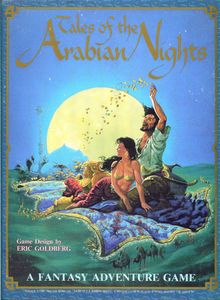The image depicts the cover of a video game titled "Tales of the Arabian Nights," prominently displayed in golden letters against a blue sky backdrop at the top. Below the title, a large moon or sun can be seen, adding an atmospheric touch to the scene. The central illustration features a man and a woman on a flying carpet, which is either purple or blue with decorative trim. The woman, with brown hair, is reclined on her side, dressed in a gold bikini top and a purple or reddish skirt. The man, who has brunette hair and is wearing an open light green or blue shirt, is kneeling behind her. Beneath the flying carpet, the background appears to be either a sky or a greenish-blue expanse that could resemble water. The bottom of the cover displays the phrase "A Fantasy Adventure Game" in white letters against a green background. In the lower left corner, it credits the game designer, Eric Goldberg. The overall scene conveys a mystical, fantasy adventure set in a mythical Arabian landscape.